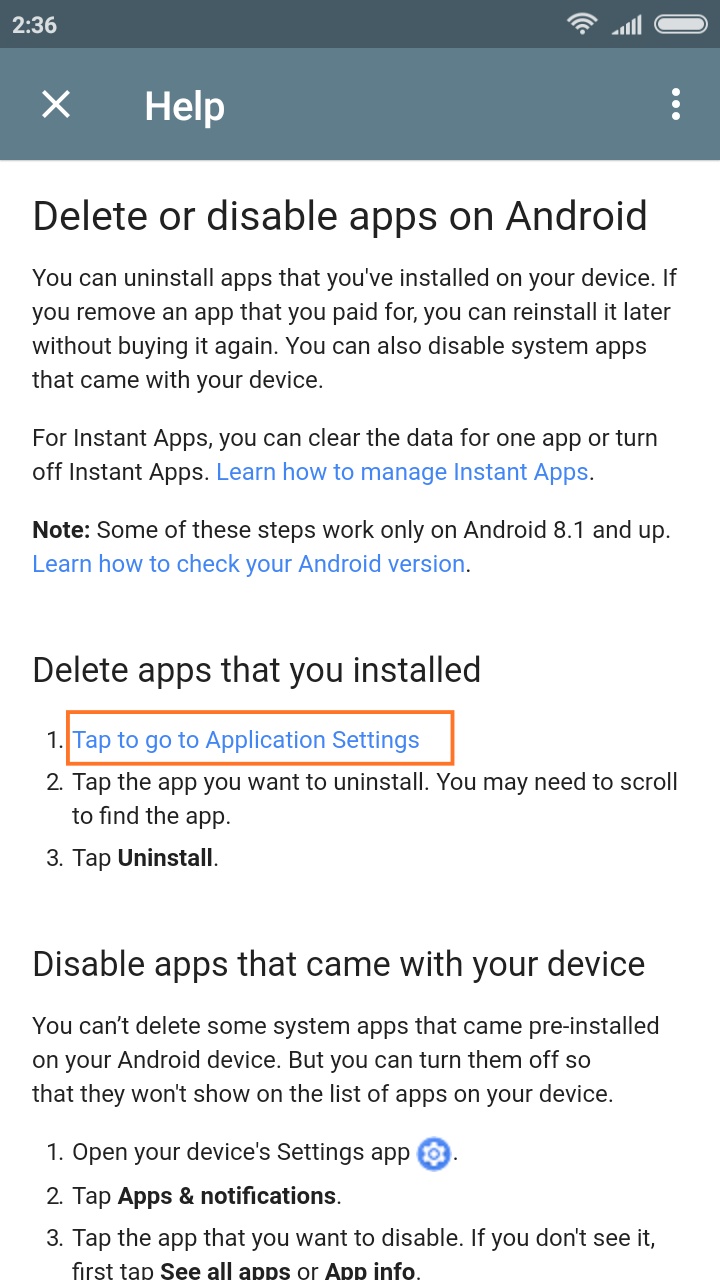Here is a cleaned-up and detailed caption for the image described:

---

Screenshot of a help article for managing an Android phone. The image is a capture from an Android mobile device. At the top of the screen, the system status bar displays the time as 2:36 on the left, and icons for Wi-Fi, mobile data, and battery life on the right. Below this, a header bar is present with the title "Help" centered, an "X" icon to close the page on the left, and a three-dot menu for additional settings on the right.

The article itself is titled "Delete or Disable Apps on Android," displayed in a grayish-blue banner. The introductory section contains a brief description and links to further help pages. Following this, the first subheading "Delete Apps That You Installed" appears, accompanied by a concise three-step process outlining how to delete installed apps. 

Another subheading, "Disable Apps That Came With Your Device," is found below, providing a brief explanation and another three-step procedure for disabling pre-installed apps. The text throughout the article is black, hyperlinks are in blue, and the background is white.